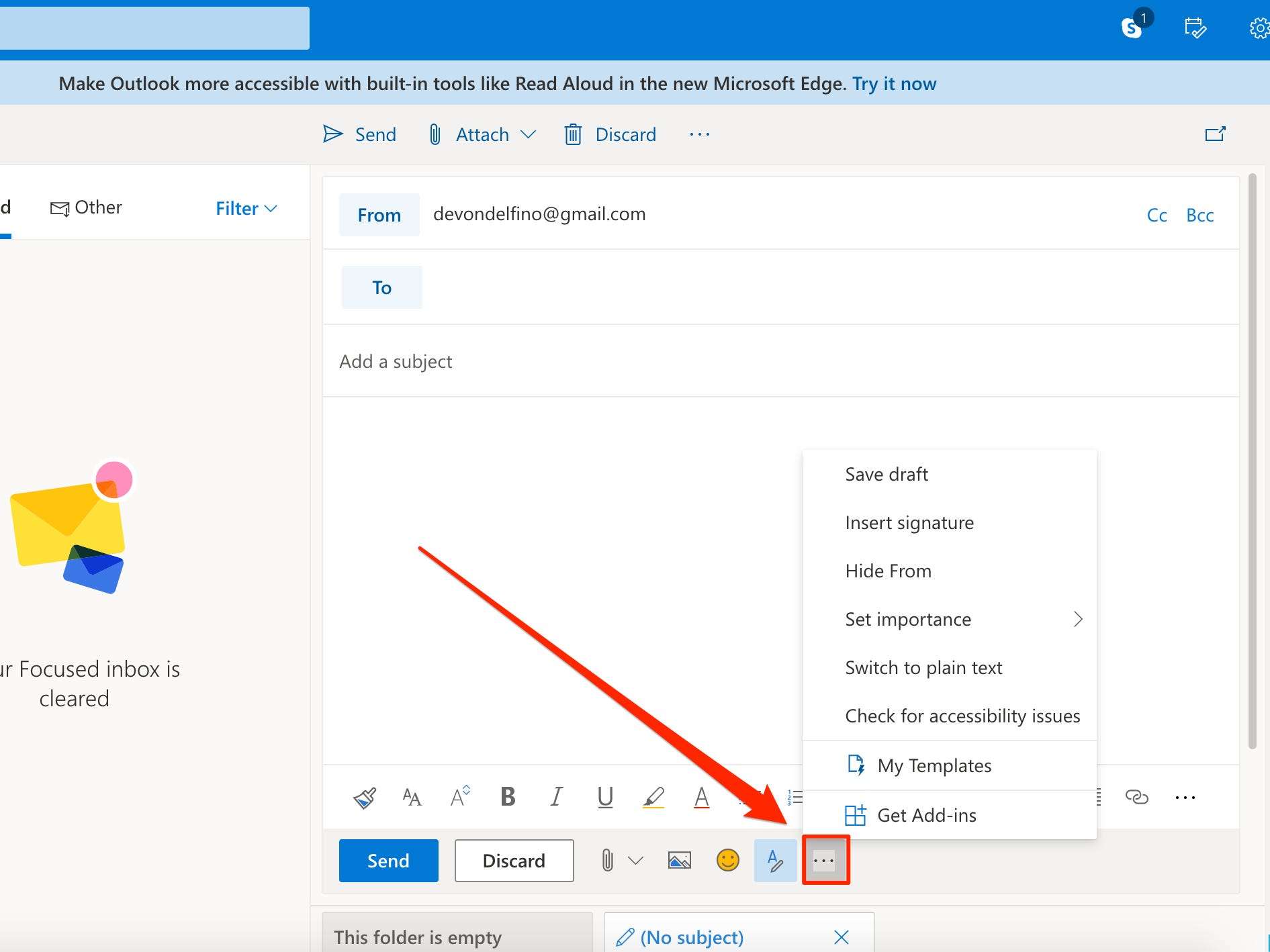The image showcases a typical email inbox interface. At the top, there's a prominent blue bar featuring a blank search bar on the left, followed by icons for Skype, a calendar with a checkmark, and a settings cog. Directly beneath this is another bar containing a message in gray text: "Make Outlook more accessible with built-in tools like Read Aloud and the new Microsoft Edge. Try it now," accompanied by a clickable blue button.

The interface includes a toolbar with icons for Send (an arrow), Attach (a paperclip), Discard (a trash can), and a menu (ellipsis). Below this, the inbox divides into two sections. The left panel contains tabs labeled "Other" and "Filter," along with a dropdown menu, with a gray section displaying icons of a yellow envelope and a blue letter.

To the right, it displays the email composition area, starting with the sender's email address, devindelfino@gmail.com. Fields for CC/BCC and the recipient's email (indicated by "To") follow. There's a field labeled "Add a Subject," next to which is a large red downward arrow pointing to an ellipsis menu, highlighting where to click. This ellipsis reveals options such as Save Draft, Insert Signature, Hide From, Set Importance, Switch to Plain Text, Check for Accessibility Issues, Align, My Templates, and Get Add-ons.

At the bottom of the composition box are formatting tools, including icons for Paintbrush, Font Size, Font Type, Bold, Italics, Underline, Marker, and Font Color (A with an underline). Further controls include buttons for Send (blue) and Discard (white), as well as icons for attaching files (paperclip), inserting images, and adding emojis. The interface ends with an empty folders section labeled "No Subject."